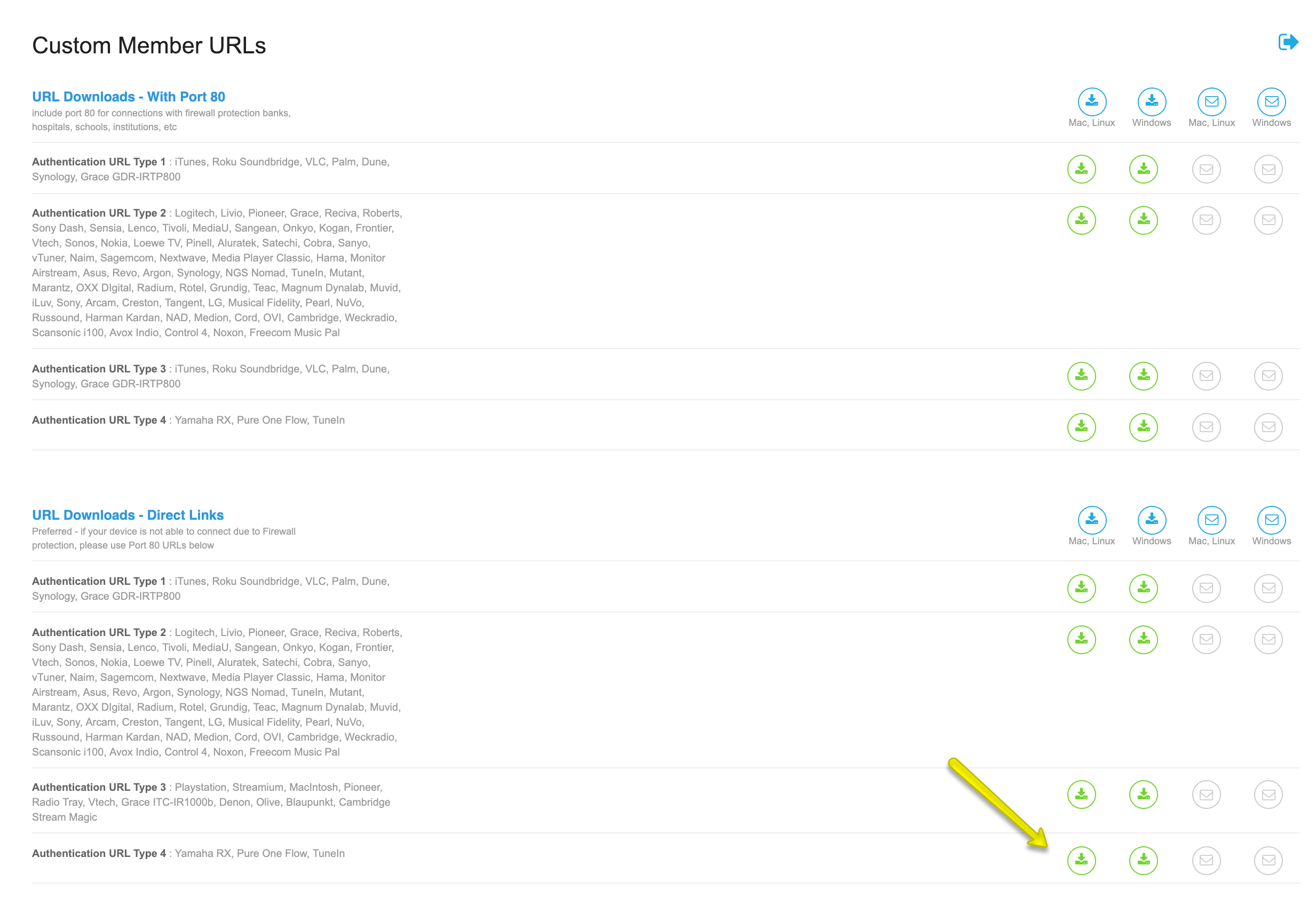In this informational image, the content is presented against a white background. On the left-hand side, text appears predominantly in black, with certain elements highlighted in blue. On the right-hand side, there are various icons corresponding to specific items listed.

Starting from the top, the first heading "Custom Member URLs" is displayed in bold black font. Directly beneath it, in blue font, it reads "URL Downloads with Port 80." Following this, there is a section of text in lighter black font.

Proceeding downward, another heading "Authentication URL Type 1" is showcased in darker black font, accompanied by additional details in smaller, light black font. Next, a section titled "Authentication URL Type 2" is shown, followed by extensive information written in a lighter gray-black font.

Continuing the list, "Authentication URL Type 3" is given in dark black font, with supplementary text in a lighter grayish-black hue. Below this, "Authentication URL Type 4" is prominently marked in dark black font, followed by extra white space.

The final highlighted item is "URL Downloads-Direct Links" written in blue font. Underneath this, there are tiny words written in light gray, providing further details in a very small font size. Each of these sections is paired with corresponding icons on the right side of the image for visual reference.